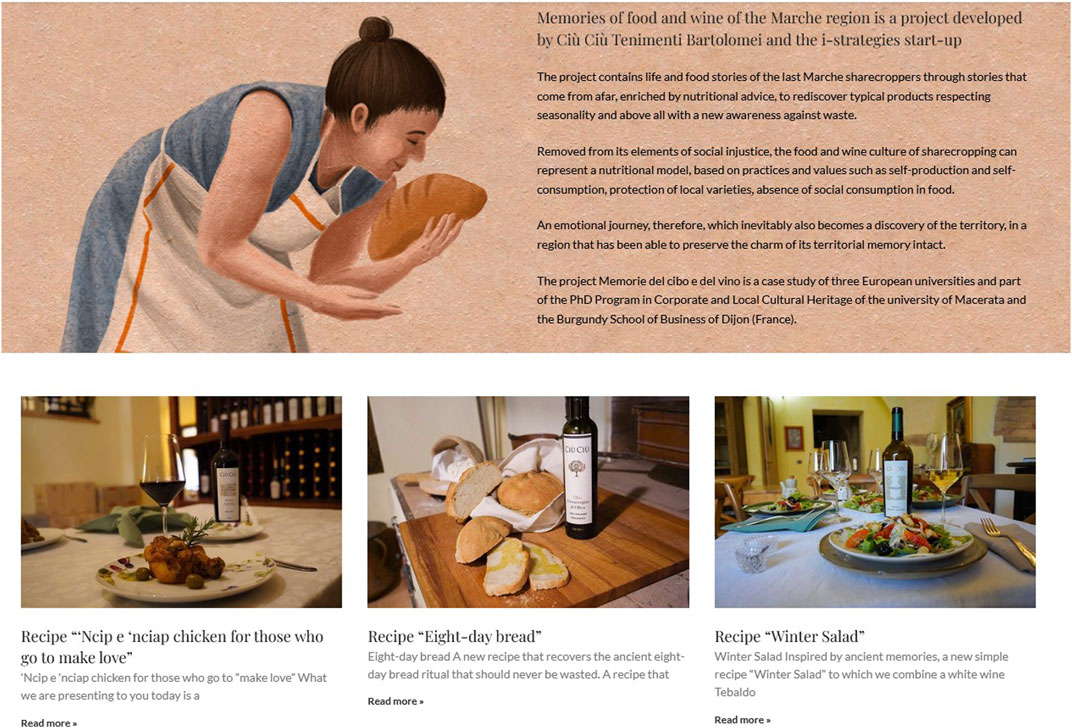The image depicts a how-to book or possibly a screenshot of a website titled "Memories of Food and Wine of the Marche Region." At the top, there is an illustration of a woman in a blue dress and white apron, her hair tied up in a bun, leaning over and cradling a freshly baked loaf of bread. The text beside her states that the project is developed by Sioux Sioux Terramente Balame and the iStrategy Startup, focusing on life and food stories of the last Marche sharecroppers, enriched with nutritional advice to rediscover typical seasonal products and promote awareness against waste.

Below the banner with the woman, there are three images:

1. A table setting with a plate of food, a wine glass filled with red wine, and a bottle of wine in the background. The caption indicates it is a recipe, possibly in French, though the exact dish is not clear.
2. A wooden cutting board with three slices of bread drizzled with olive oil, accompanied by a basket of bread and a bottle of wine. The caption reads "Recipe 8 Day Bread."
3. A plate of winter salad alongside a glass of white wine and a bottle of wine. The caption reads "Recipe Winter Salad."

The project aims to capture the essence of the Marche region's culinary heritage through evocative imagery and traditional recipes.